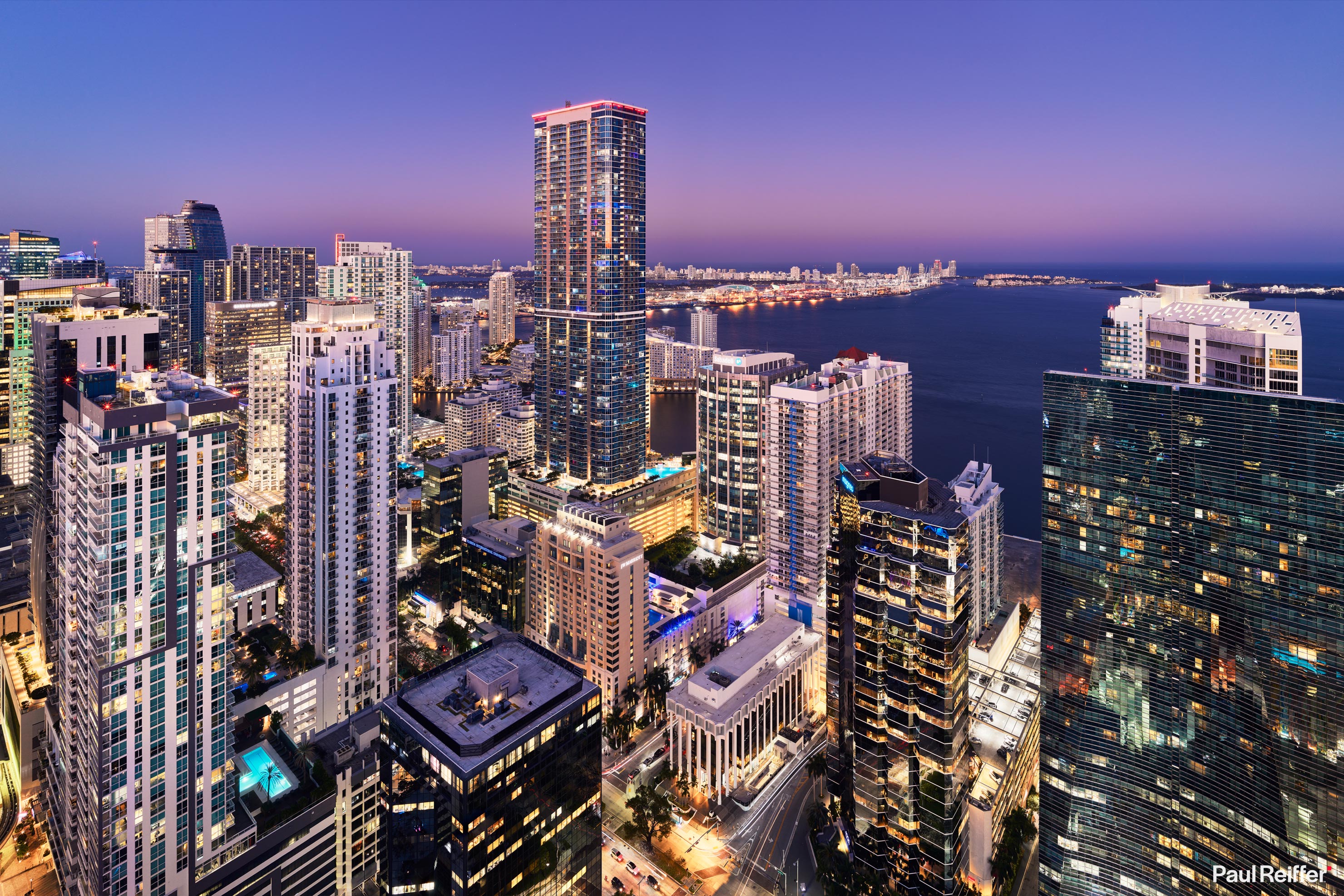This image is a high-angle, likely drone-captured photograph of a bustling waterfront cityscape during early evening. The sky is a blend of purple and light blue hues, occupying the upper fifth of the image, and casting a serene glow over the scene. Dominating the view are numerous tall skyscrapers, some towering up to 100 stories, primarily in shades of gray, white, and black, interspersed with vibrant colors like blue, orange, and green. Many of the buildings are made of glass and are brightly illuminated, their lights twinkling against the dimming sky as night approaches. In the lower right-hand corner, the image features the superimposed text "Paul Reifer," indicating the commissioner's credit. In the distance, the ocean meets the city, dotted with boats, adding a tranquil counterpoint to the urban complexity. The angle of the shot allows a clear view of the rooftops and a glimpse of the streets below, further emphasizing the density and intricacy of this metropolitan area.